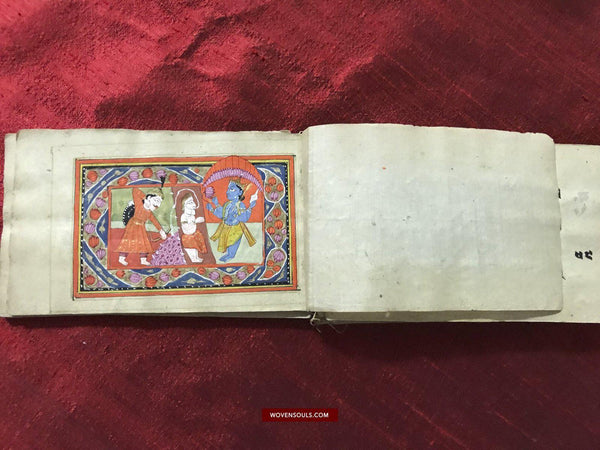This detailed photograph captures an open, old paper-bound book placed on a textured red silk tablecloth. The book appears handmade, suggested by its unevenly sized pages and the visible threading, indicating either cloth or heavily wrinkled paper. The photograph prominently features an intricate illustration bordered in red and gold. The artwork, done in vibrant reds, purples, greens, and yellows, depicts various characters with a backdrop of a blue, orange, and light green design. 

On the left, there is a depiction of a figure in a red long-sleeved top and skirt, with one arm extended downward towards some pink flowers while their other arm is cocked with a fist. The central character, possibly representing a deity like Shiva, boasts purple or blue multi-armed imagery with a yellow sash around the waist and is surrounded by red and purple stone-like fixtures encircled by green. The right side showcases a blue-skinned figure with a crown and a gold skirt, appearing to hold or juggle something. The fabric background adds a rich texture to the composition, enhancing the overall vintage and sacred aesthetic of the scene. At the bottom of the image, "wovensouls.com" is inscribed in white text.